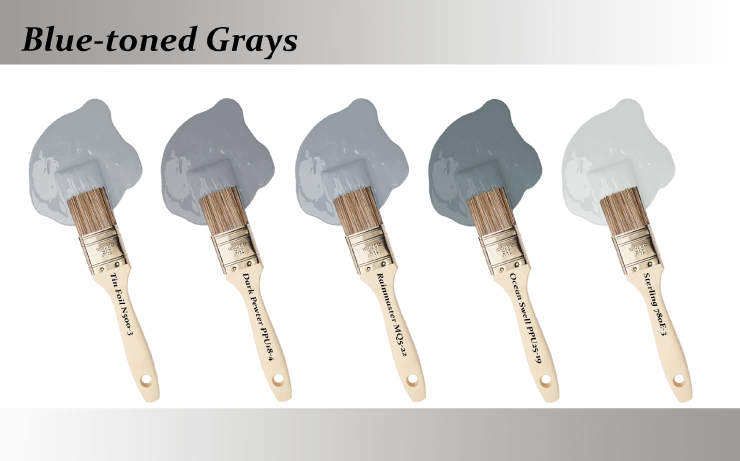The image showcases five paintbrushes with wooden handles that are a light off-white color, each imprinted with small, black text. The brush handles read, from left to right, 'Sterling,' 'Ocean Swell,' 'Ruminator,' 'Dark Pewter,' and 'Tinfoil.' These paintbrushes also feature a hole at the bottom of each handle. The top part of the brushes, where the fibers are, is made of metal, and the bristles are gray but dipped in various shades of paint that range from light gray to almost black, to slightly lighter gray, to a green-toned cement color, and finally to white. Above the paintbrushes is a gray bar containing the text 'Blue-Toned Grays,' and below them, another empty gray bar frames the image. This minimalistic setup highlights the different shades of blue-toned gray paints, emphasizing the variations in color against a plain white background.